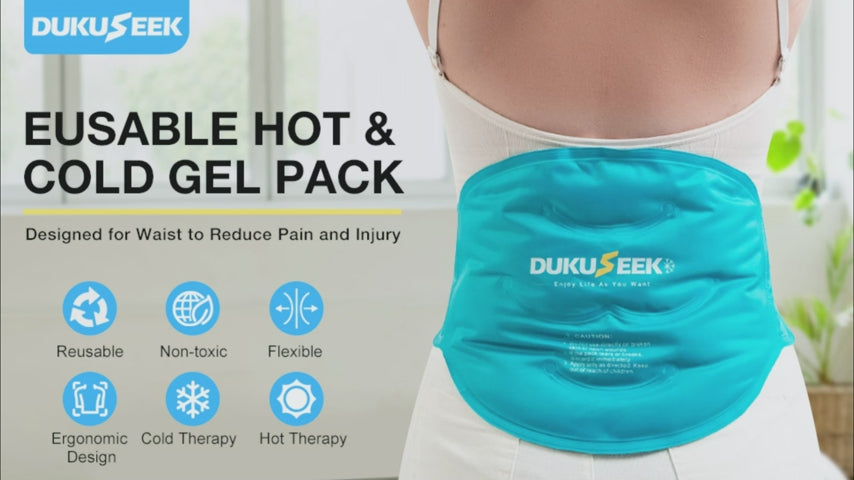This advertisement showcases a product called DookuSeek, specifically an E-usable Hot and Cold Gel Pack designed for pain relief and injury prevention. The ad is horizontally oriented, featuring a woman in a white camisole and jeans with the blue gel pack wrapped around her waist and lower back. The DookuSeek logo is prominently displayed on the pack, with the capital "S" in yellow and the other letters in white.

The left side of the image details the product's benefits, highlighted by six blue circular icons each containing simple graphics: 
1. Reusable (represented by rotating arrows),
2. Non-toxic (depicted as the Earth with a leaf),
3. Flexible (shown with a line and bidirectional arrows),
4. Ergonomic Design (illustrating a back with directional arrows),
5. Cold Therapy (marked by a snowflake),
6. Hot Therapy (represented by a sun).

Additionally, beneath a yellow dividing line, bold black text states, "designed for reduced waist pain and injury," emphasizing the product's purpose. The setting includes a white room with windows and green potted plants, enhancing the clean and sleek aesthetic of the ad.